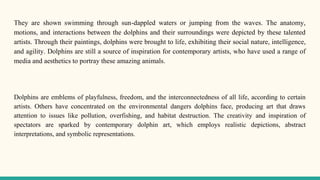This image captures an excerpt from a text, likely from the inside of a book, set against a cream-colored background with black print. At the bottom, there is a touch of green or aquamarine color. The text describes how dolphins are depicted swimming through sun-dappled waters or leaping from the waves. These talented artists illustrate the anatomy, movements, and interactions between dolphins and their environment, bringing them to life and showcasing their social nature, intelligence, and agility. Contemporary artists continue to find inspiration in dolphins, utilizing various media and aesthetics to portray these remarkable creatures. The second paragraph of the text explains that dolphins symbolize playfulness, freedom, and the interconnectedness of life to some artists. Others focus on the environmental threats dolphins face, such as pollution, overfishing, and habitat destruction, creating art to highlight these critical issues. The creativity of contemporary dolphin art includes realistic depictions, abstract interpretations, and symbolic representations, engaging and inspiring a broad audience.